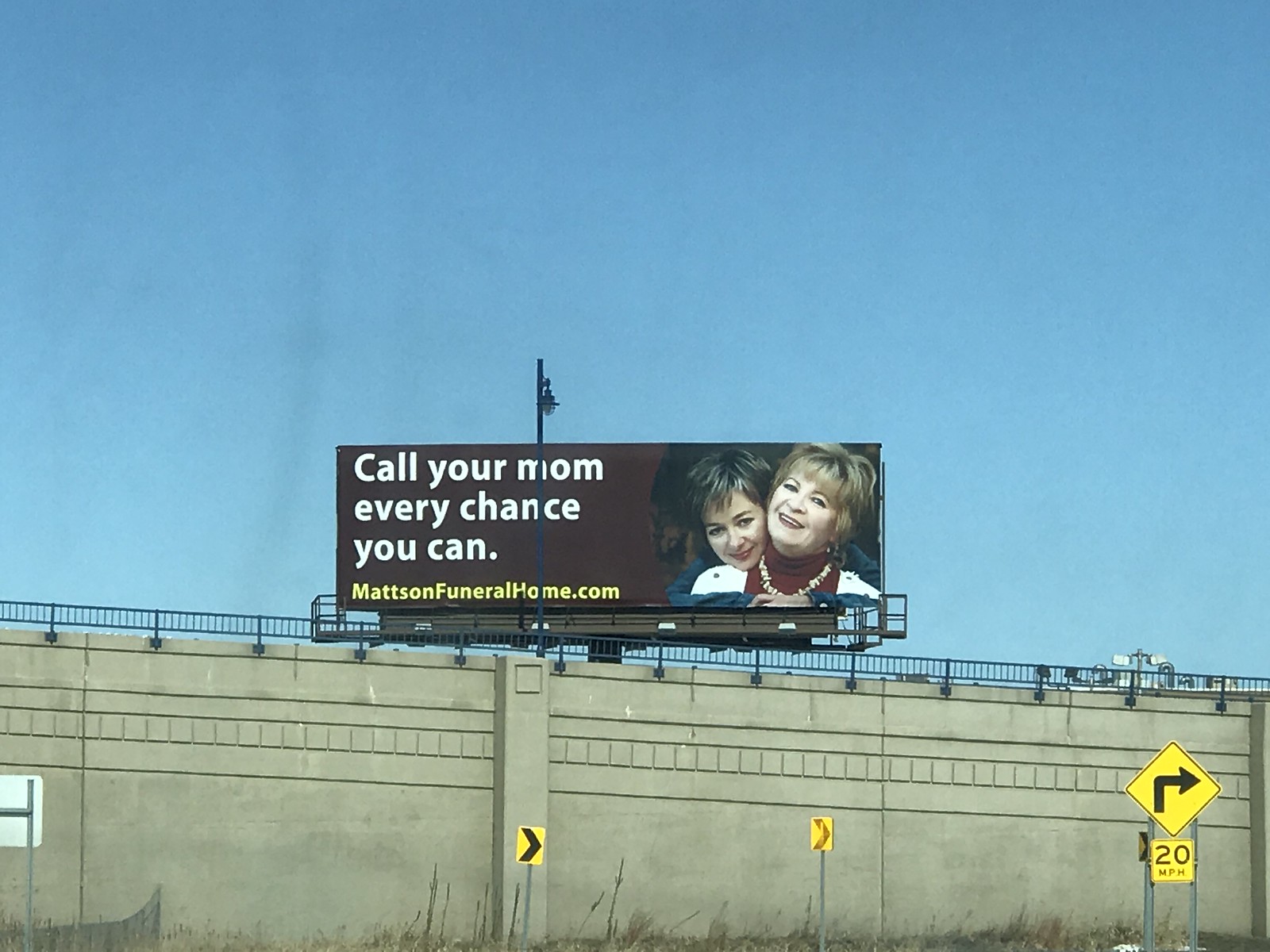This detailed color photo captures a large, rectangular billboard positioned above a substantial, dark gray concrete retaining wall with a black railing, alongside a freeway. The billboard, which features a chocolate brown background, prominently displays the text "Call your mom every chance you can" in white. Below this message, "mattsonfuneralhome.com" appears in yellow. The right side of the billboard includes a small rectangle containing an image of two women embracing—likely a mother and daughter. The older woman on the right, sporting lighter-colored, short blonde hair, is adorned in a red turtleneck, a chunky necklace, and a white coat. Hugging her from behind is a younger woman with darker brown hair, dressed in a blue long-sleeved top. Below the retaining wall, there are several yellow signs with black arrows pointing to the right, and a rectangular sign indicating "20 MPH." The photo was taken outdoors, under a clear blue sky, adding a sense of everyday reality to the poignant billboard message.